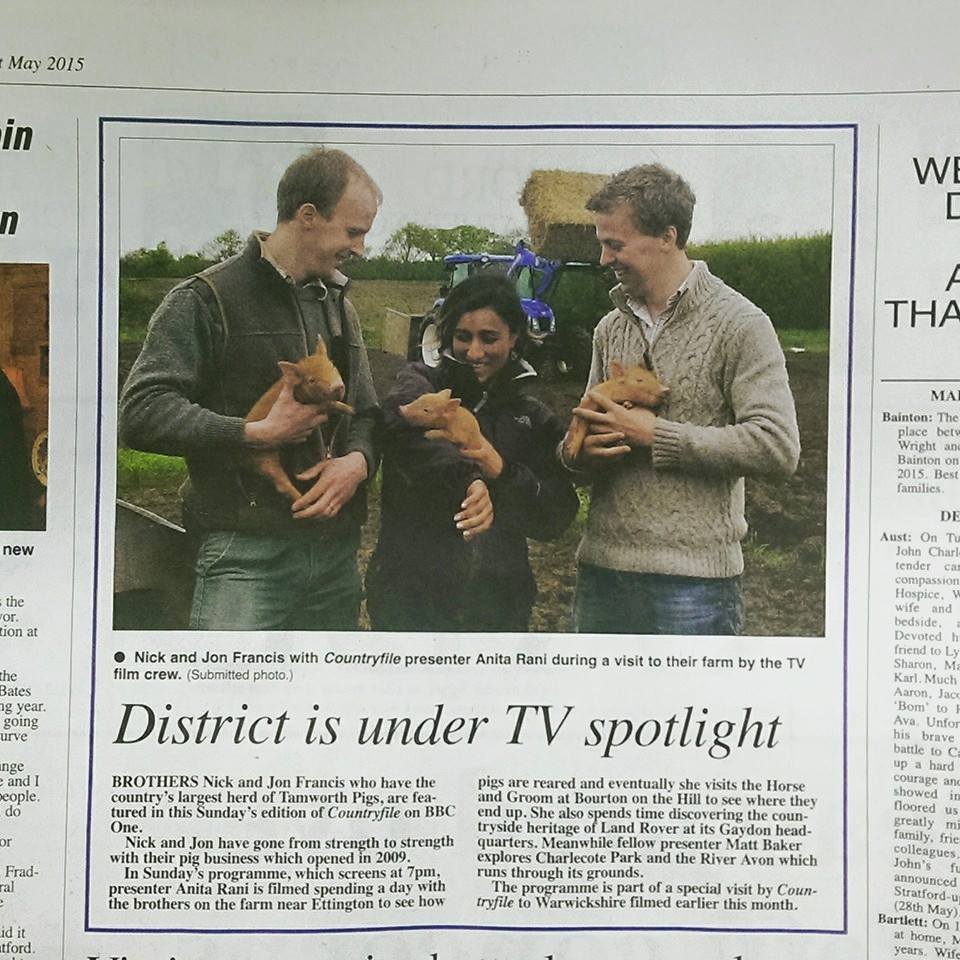In the photograph accompanying the newspaper article, three individuals—two men and a woman—delightfully cradle small piglets, each roughly the size of a loaf of bread. The men are identified as Nick and John Francis, alongside Country File presenter Anita Ronnie. The image captures a moment from a visit to their farm by a TV film crew. The headline of the article reads, "District is under TV spotlight."

Brothers Nick and John Francis, proud owners of the country's largest herd of Tamworth pigs, are featured in the upcoming Sunday edition of Country File on BBC One. Since launching their pig business in 2009, the brothers have achieved considerable success. The program, airing at 7pm, follows presenter Anita Ronnie as she spends a day at their farm near Eddington, gaining insight into pig rearing. Her journey concludes at the Horse and Groom in Borton-on-the-Hill, where she learns about the final destination of the pigs.

Additionally, the episode showcases Anita exploring the countryside heritage of Land Rover at its Graydon headquarters. Meanwhile, fellow presenter Matt Baker visits Charlecote Park and the River Avon, immersing viewers in the natural beauty of the grounds. This episode is part of a special feature by Country File, highlighting various locations across Warwickshire and filmed earlier this month.